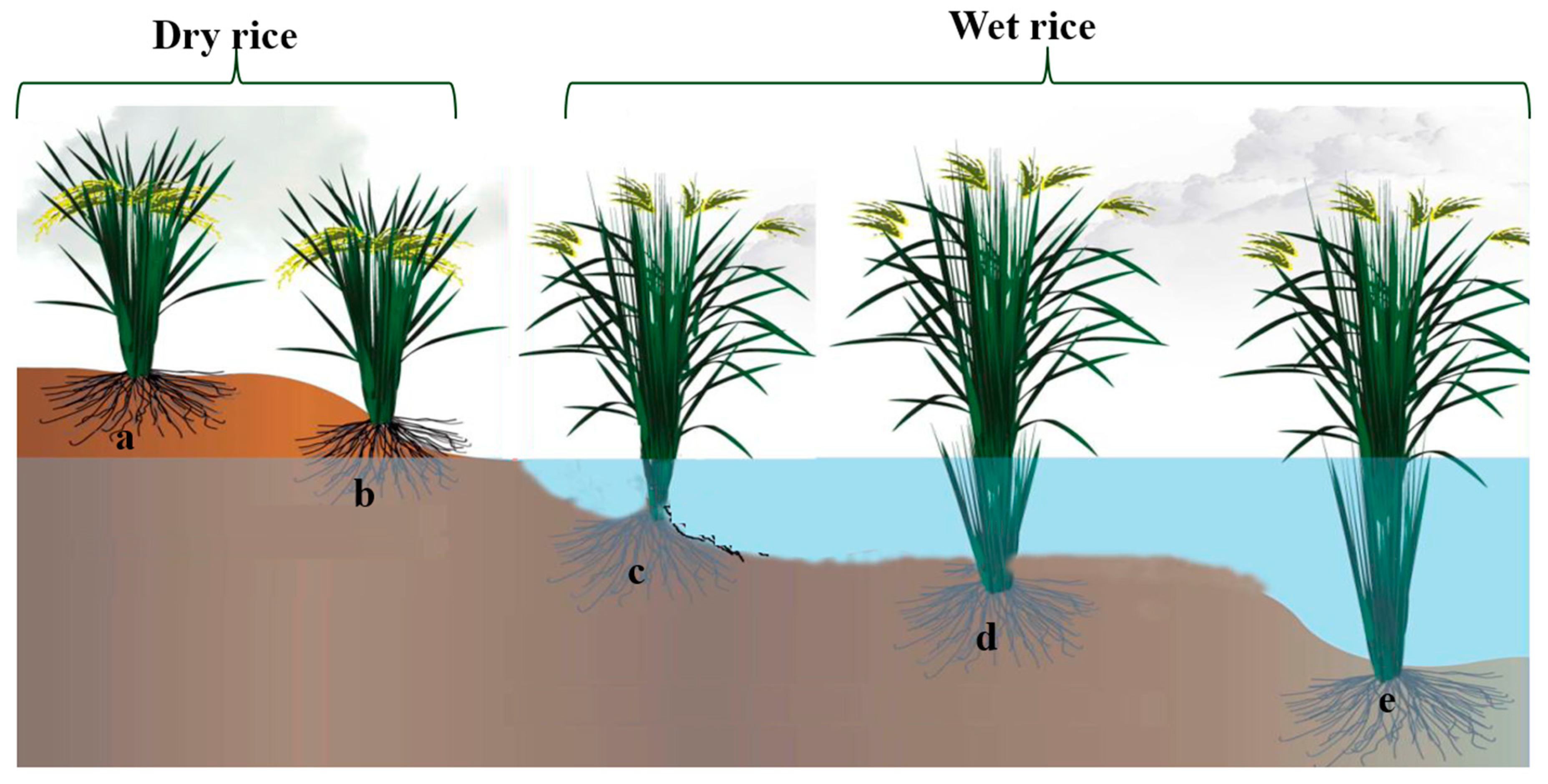This image is a detailed graphic presenting the different growth stages of rice crops, categorized into dry and wet rice stages. A waterline runs horizontally through the center of the image, with the lower half tinted blue to represent water, and the upper half shaded white, symbolizing the sky. Five rice plants are depicted and labeled A, B, C, D, and E from left to right.

On the left side, A and B represent the dry rice stage and are situated above the waterline on orange-brown soil. Plant A is the smallest, and Plant B is slightly larger, showing the early growth stages of dry rice. These plants are marked with the text "dry rice."

Moving rightward, C, D, and E illustrate the wet rice stage, where the plants are increasingly submerged underwater. The soil here slopes below the waterline. The plants in this section grow progressively taller from C to E, with E being the tallest. The text "wet rice" labels this section.

All the plants are green with yellow seed clusters at their tops. The background features a faint depiction of clouds, adding to the overall visual detail. This graphic effectively demonstrates the various environmental conditions and growth stages of rice plants—from dry soil to submerged aquatic environments.